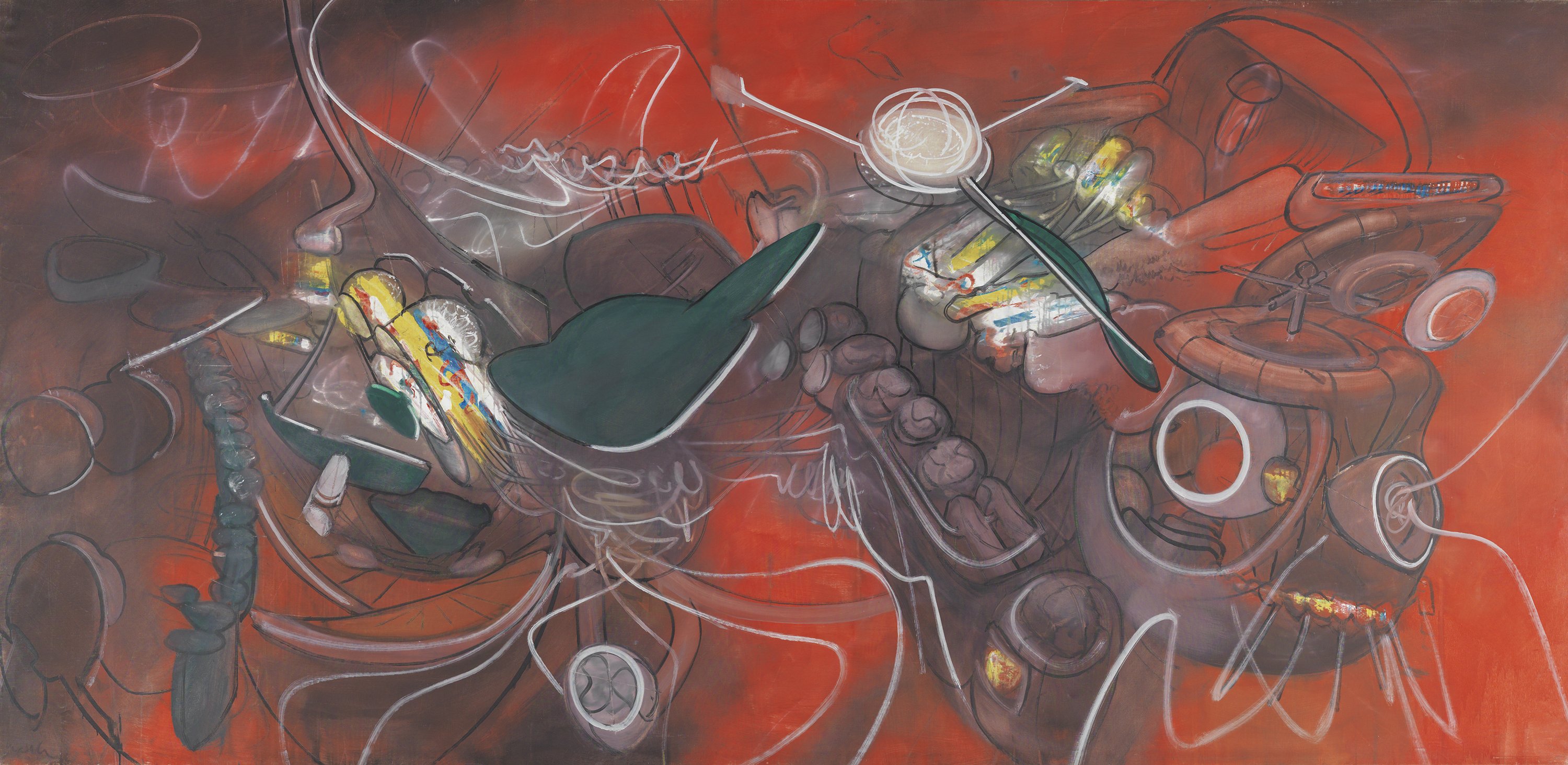The image is a highly detailed abstract painting with a red dominant background enhanced by vibrant splashes of whites, purples, and other colors. The composition primarily features rough and chaotic lines resembling graffiti or spray paint, intertwined with geometric shapes and robotic elements. Notable in the top right corner is an outline of a sofa, while the left side shows what could be an end table or barrel with a circular hole. The foreground includes a faint outline of a chair and possibly more indistinct structures. The painting is infused with white lines and strokes creating an impression of electrical energy or graffiti overlays. Yellow and blue blotches add to the complexity, especially in the left corner. The overall aesthetic is a mixture of mechanical forms and abstract elements, making it an intriguing, though challenging, piece to define precisely.